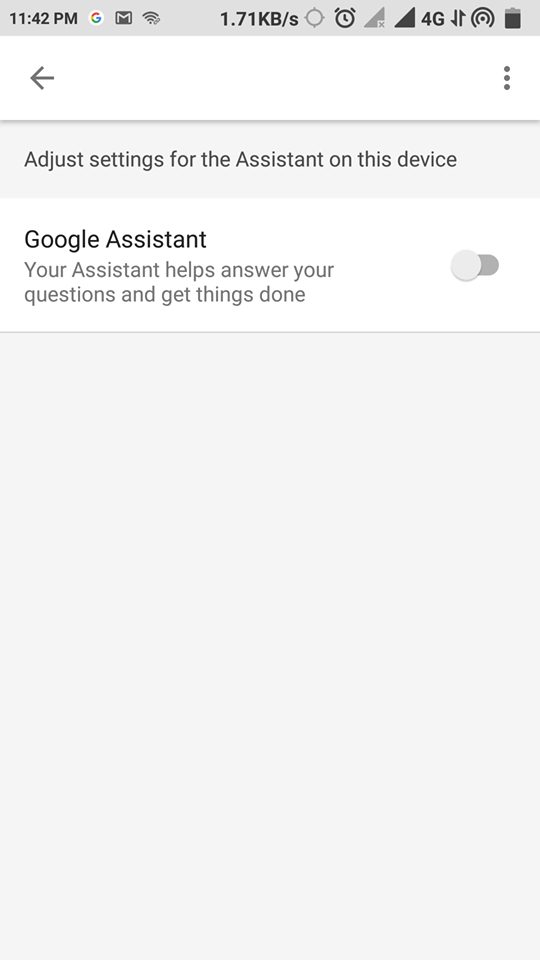This image depicts a mobile device displaying a settings page. At the very top of the screen, various status icons are visible, including the current time, a Google icon, a battery percentage indicator, a 4G signal strength icon, and a stopwatch icon. Directly below these icons, there is a grey back arrow and a grey three-dot menu symbol. The primary text on the screen reads: "Adjust settings for the assistant on this device," followed by a prominent title, "Google Assistant." Below this, a descriptive text explains, "Your assistant helps you answer questions and get things done."

A grey toggle button is present, typically used to indicate whether the setting is turned off or on. The overall design of the page features a grey and white color scheme with black text. The majority of the screen is framed by a grey border, while the specific sections containing text have a white background, allowing the black and grey text to stand out clearly. This layout resembles a typical settings page on a smartphone where users can customize features like the Google Assistant.

Additionally, a few more logos are situated at the top of the screen. Centered on the display, there is a data indicator reading "1.71 kb/s," which likely represents the WiFi network's upload speed.